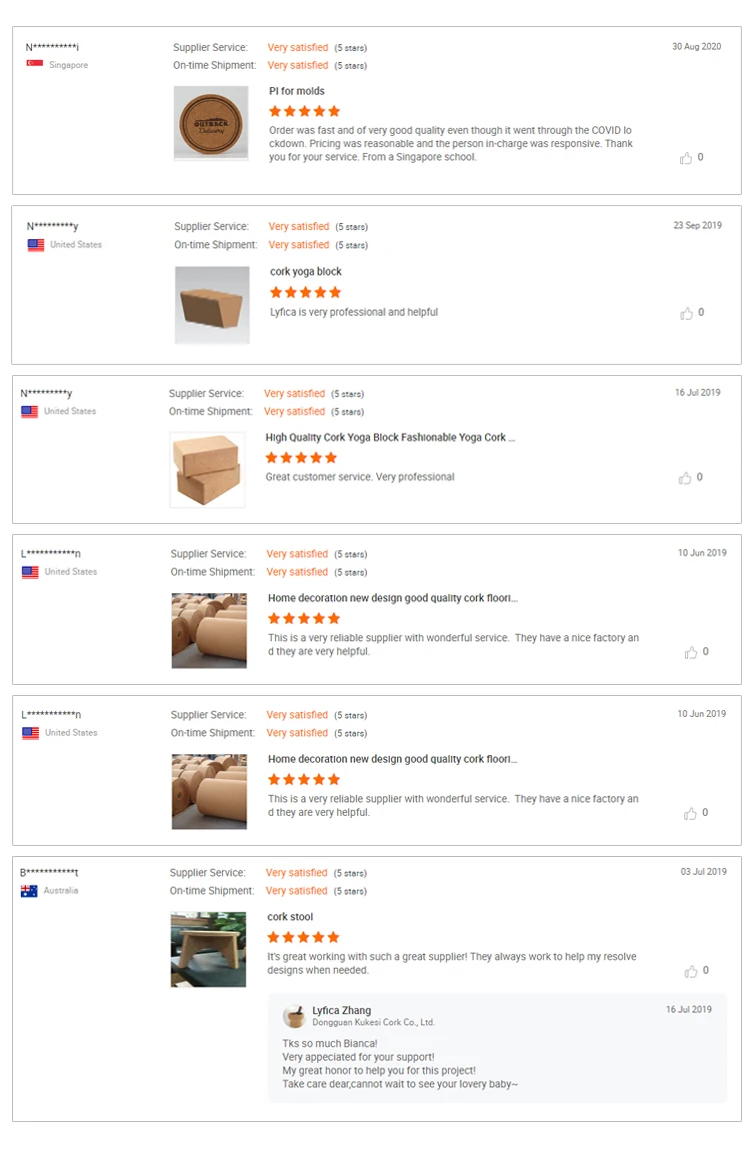The image appears to be a detailed product review on a white backdrop, similar to those found on e-commerce websites. The composition includes various sections and numerous text boxes.

At the top, there's a box with unreadable black text, followed by another red box with "Singapore" beside it. Next to this, it says "Supplier Service." Just below, "On Time Shipment" is mentioned.
  
Moving further down, the phrase "Very Satisfied" is repeated twice with "Five Stars" above each instance.

There is a box containing an image of a circular brown object. Adjacent to it, text reads:

"Order was fast and of very good quality even though it went through the COVID crackdown. Pricing was reasonable, and the person in charge was responsible. Thank you for your service from a Singapore school."

Below this, there is a picture of a brown loaf with the text:

"Lifca is very professional and helpful."

Next to that is an image of two brown boxes with the label:

"High Quality Quark Yoga Block and Fashionable Yoga Quark."

Below this, it says:

"Great Customer Service, Very Professional."

Following this, there's a picture of several rolled up brown mats alongside text stating:

"Home Decoration, New Design, Good Quality Quark something."

Underneath, it notes:

"It was a very reliable supplier with wonderful service. They have a nice factory and they are very helpful."

Below is another picture of multiple rolled up brown rugs with adjacent text that again claims:

"Home Decoration, New Design, Good Quality Quark something."

Further down, there is an outdoor image featuring a brown bench with the following text:

"Quark Stool"

There is also some black text that is not clearly readable, seemingly stating:

"It's great working with such a great supplier."